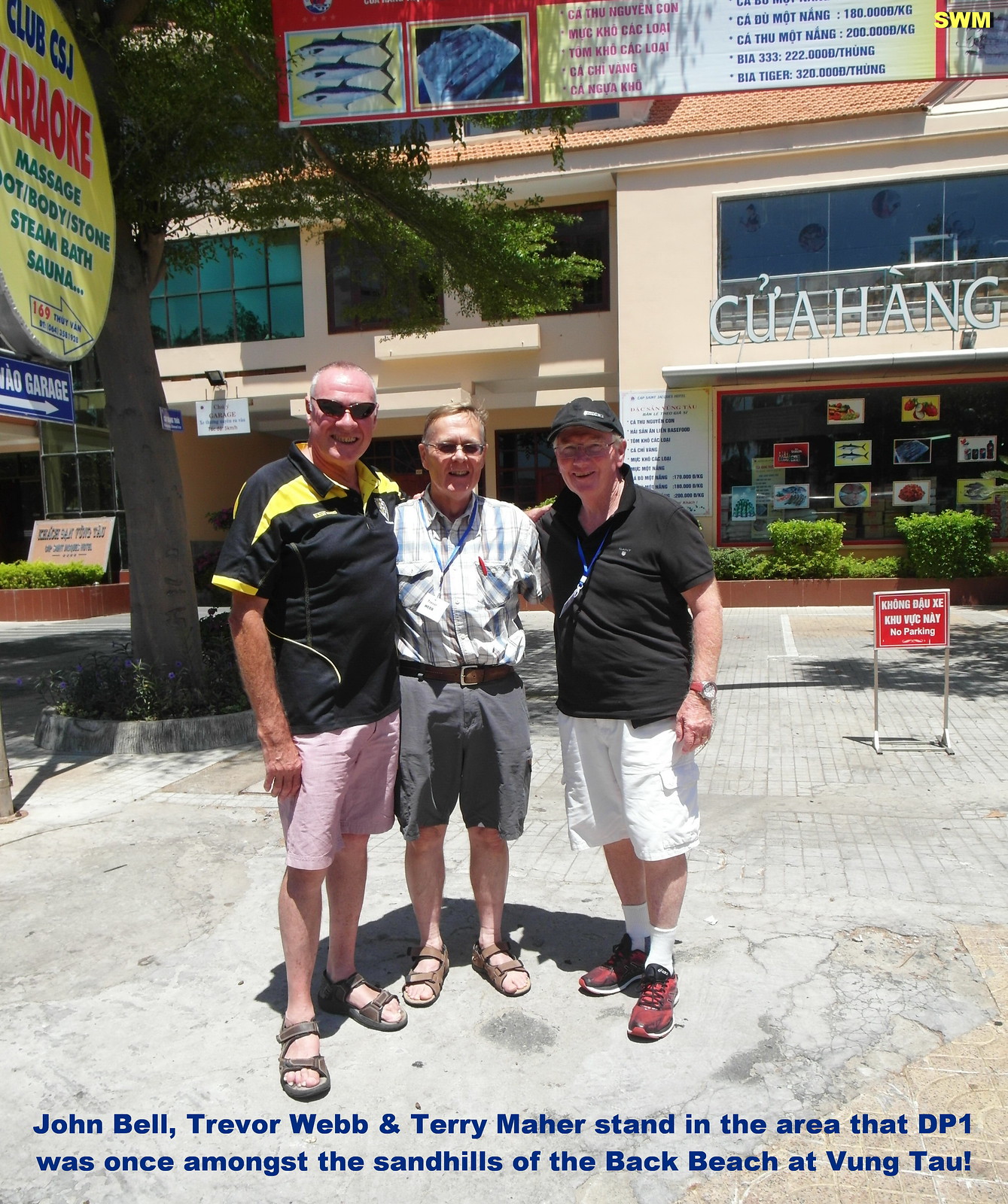This vibrant color photograph captures three older men, identified as John Bell, Trevor Webb, and Terry Marks, standing in a plaza surrounded by buildings. The setting appears to be in Vung Tau, Vietnam, indicated by the signage and caption. The men, who are likely in their 60s, are casually dressed in short-sleeved shirts and shorts; two are wearing sandals while the third has on sneakers and a baseball cap. John Bell is in a black and yellow shirt with pink shorts, Trevor Webb sports a white and blue plaid shirt with gray shorts, and Terry Marks dons a black shirt with white shorts. Two of them wear sunglasses, while the other has regular glasses. Behind them, there are multiple signs in Vietnamese, with one prominently advertising karaoke for Club CSJ, as well as massage, steam bath, and sauna services. Additionally, a storefront sign reading "Cua Hang" (Quahag), is visible. A tree is also situated to the left side of the men in the background. The caption at the bottom of the photograph notes that these three men are standing in an area that used to be the site of DP1 amongst the sandhills of the back beach at Vung Tau, adding historical significance to their visit.